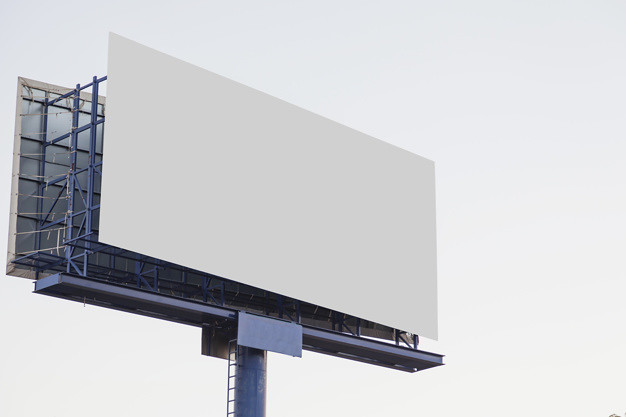The image captures a large, two-sided, blank billboard set against a flat, grayish-white sky. The billboard, primarily beige, reveals no graphics or text, thus appearing completely empty. It is supported by a sturdy metal structure comprising a grid of horizontal and vertical steel beams. The metal frame, bluish in the light, includes scaffolding and a prominent cylindrical support column equipped with a ladder. At the top of this column, a bracket secures the dual-sided advertising faces of the billboard. A dark gray base anchors the entire structure, complemented by square or rectangular metal rails running parallel underneath the billboard. The left edge of the billboard's backside is faintly visible, peeking from behind.